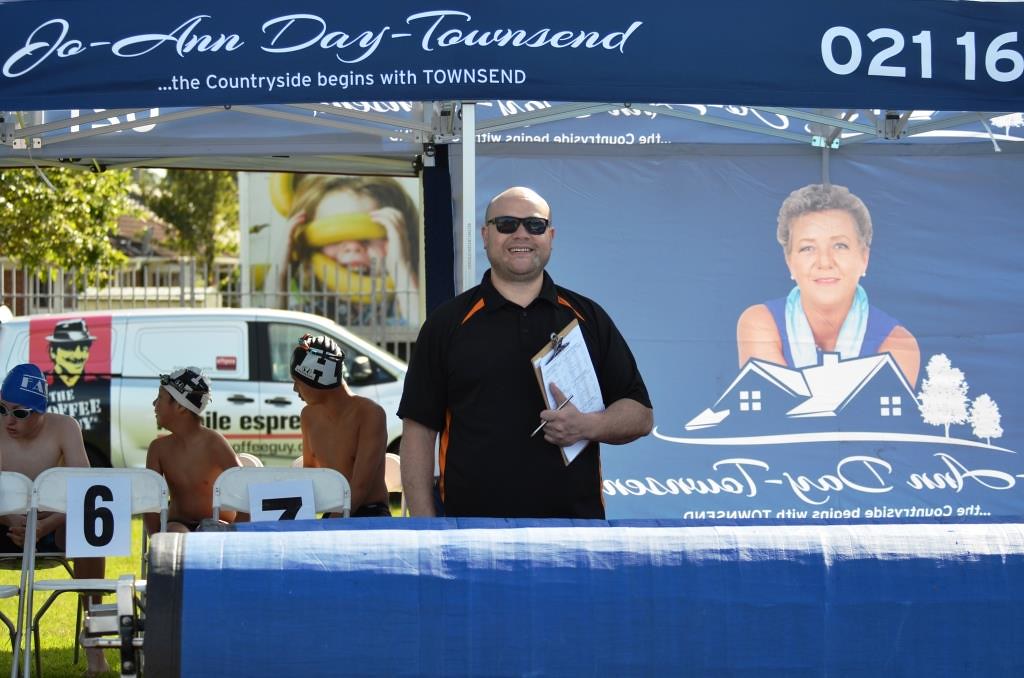In the image, a man is seen standing behind a table covered with a blue tarp, under an open-sided canopy tent, suggesting an outdoor event setting, possibly a triathlon. He's visible from the waist up, wearing a black collared polo shirt with orange shoulder stripes, and sporting black sunglasses. In his left hand, he holds a brown clipboard with a metal clip and unreadable printed text, along with a gray pen. The backdrop features advertisements and a banner reading "Joe Ann Day Townsend," accompanied by the partial number "02116." This banner also displays an image of a woman looking over a house rooftop, hinting that Joe Ann Day Townsend, likely a realtor, is sponsoring the event. To the left, three males wearing swim caps and trunks sit on numbered chairs, indicative of participants in a swimming event.